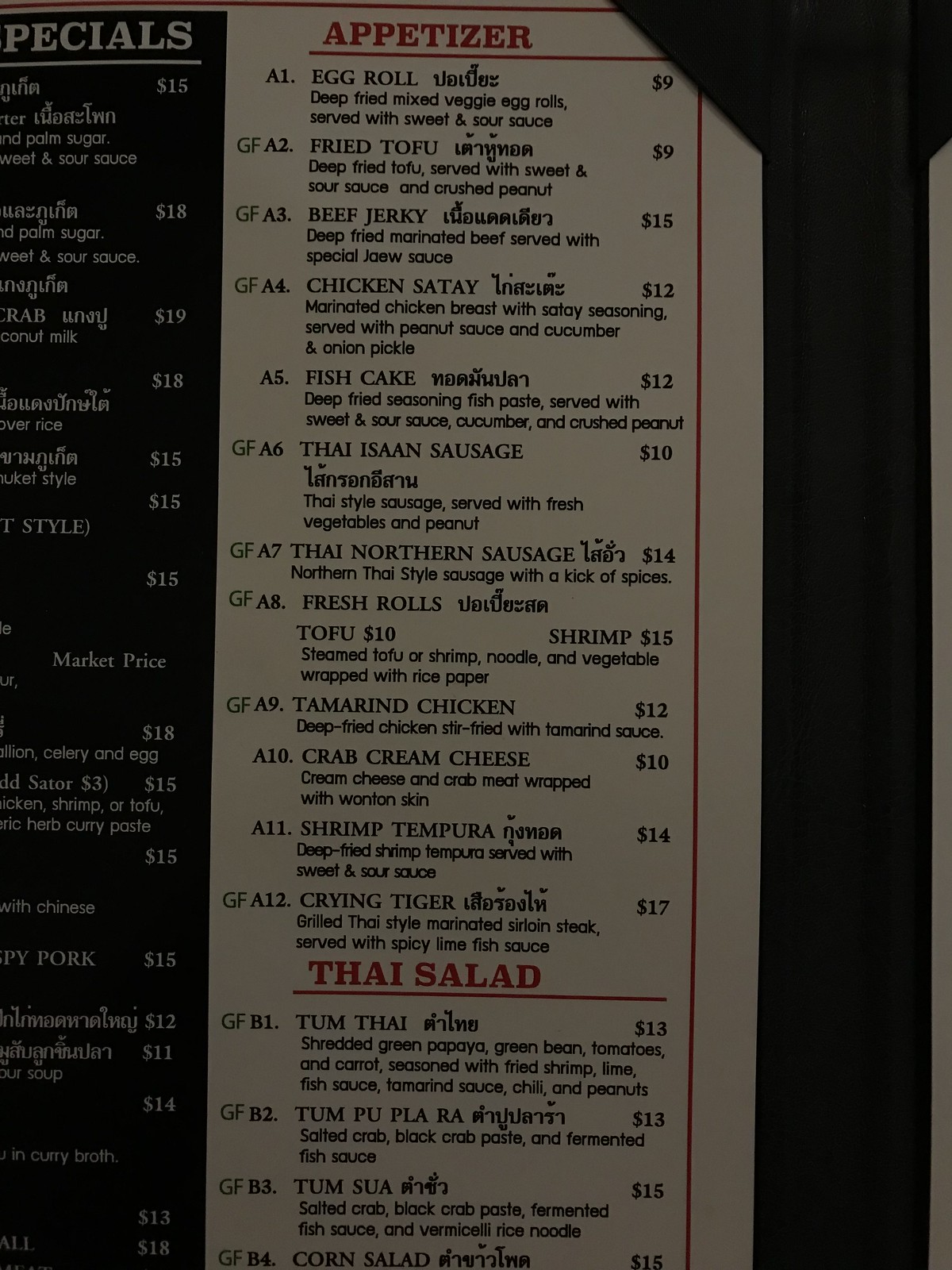The image features a vertically-oriented rectangular menu, closely zoomed in to capture intricate details. On the right-hand side of the image, there's a narrow white strip, possibly indicating the menu's edge, adjacent to a darkish brown area that could be part of a table, although it’s not clear. The lighting is dim, but discernible elements of the menu stand out.

On the right side, the menu has a black section, but it's partially cut off. Only part of the word "SPECIALS" is visible, specifically the letters "P-E-C-I-A-L-S," along with partial descriptions and price details, some of which are presented in English and another language using distinct symbols.

The left side of the menu is completely visible and features a white background with "APPETIZER" prominently displayed in red, underlined and framed with red lines. Listed items include "Egg Roll" and "Fried Tofu," each accompanied by its name in another language, a brief description, and its price. The menu items are arranged vertically, providing a structured overview as one reads downwards.